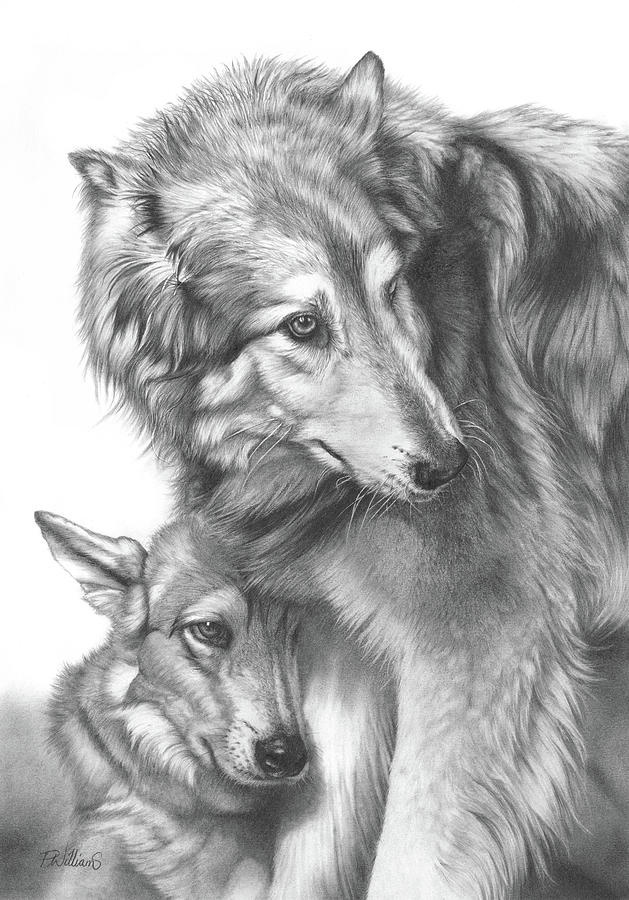This black and white etching meticulously captures two wolves in a protective, affectionate pose. The larger wolf, presumably the mother, stands tall with a sheltering posture, her smaller ears and lighter-colored eyes attentively gazing to the right. The younger wolf, with its larger ears and dark eyes, leans against her leg, nuzzling into her fur in a sign of comfort and closeness. The intricate detailing emphasizes the texture of their fur, with each strand distinctly etched to convey depth and realism. Although the wolves are uncolored, the shading masterfully brings out the contrasts in their fur and the tender dynamics of their interaction. The artwork is signed in the bottom left corner, though the name is difficult to decipher, potentially reading "P. Williams."